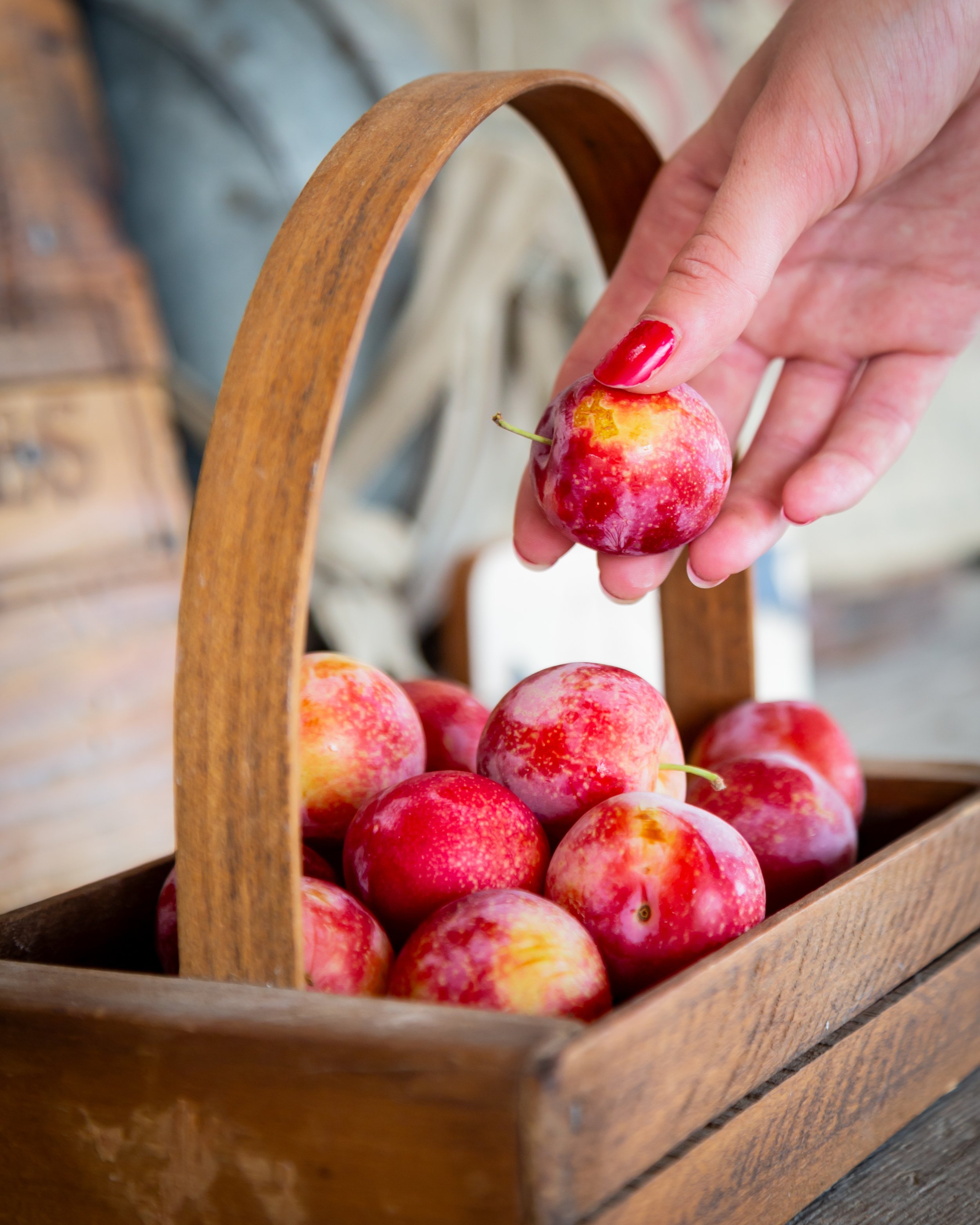This image depicts a farmer's market scene focused on a sturdy, brown wooden basket filled with approximately ten small, red and yellow peaches. The basket, which features a handle arching over its middle, sits prominently in the center of the shot. The background is blurred, suggesting a bustling market stand. In the top right corner, a white-skinned hand with long, red-manicured nails, one of which is chipped on the thumb, is seen either placing or removing a peach from the basket. The peaches have a slight dusty coating and vary slightly in red and orange hues. The perspective of the photograph is almost level with the basket, highlighting the details of both the fruit and the hand interacting with them.